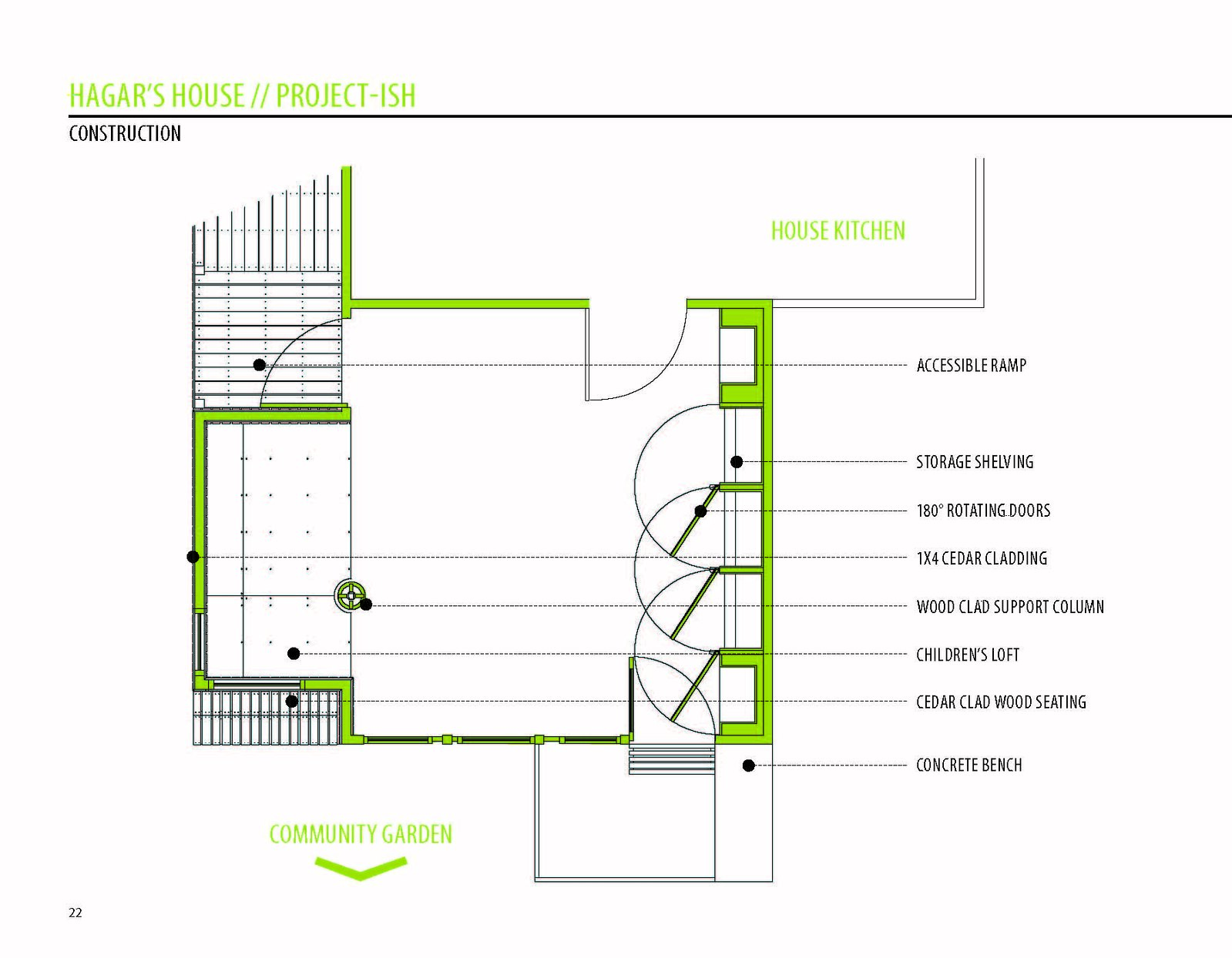The image is a detailed architectural drawing set against a white background. At the top, there is a black border line above which the title "Hager's House // Project-ish" is printed in green, uppercase letters. Below the black dividing line, the word "CONSTRUCTION" is displayed in black, uppercase text on the left-hand side.

The drawing itself appears to be a top-down view of a house layout. Key areas and items within the layout are labeled, with most descriptions positioned on the right side in black print. These labels include: "accessible ramp," "storage shelving," "180-degree rotating doors," "one-by-four cedar cladding," "wood-clad support column," "children's loft," "cedar-clad wood seating," and "concrete bench." The layout also features numerous squares and rectangles, some outlined in the same green color as the title and the label "house kitchen," which is located in the upper right part of the drawing.

Additionally, the lower left corner of the layout includes the label "community garden" with an arrow indicating its placement outside of the house. The diagram also shows various doorways with their swinging angles, and different room dividers, contributing to the comprehensiveness of this architectural blueprint.